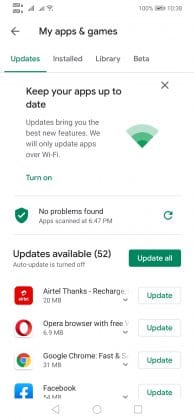The screenshot depicts a mobile phone screen, specifically in the "My apps & games" section within the Settings menu of the Google Play Store. Positioned at the upper-right corner, the phone shows a time of 10:39 and indicates a battery level of 10%. The screen under "My apps & games" features four clickable tabs aligned from left to right: Updates, Installed, Library, and Beta. The "Updates" tab is highlighted in green.

Directly below this tab, a message advises users to "Keep your apps up to date," with an option to enable automatic updates. Scrolling down further, there are icons representing four apps that need updates: Airtel Thanks, Opera Browser, Google Chrome, and Facebook. Each app is listed with its respective icon and name, accompanied by an individual "Update" button. Additionally, a green "Update all" button is prominently displayed above the list of apps.

The screen headline indicates that there are a total of 52 app updates available.